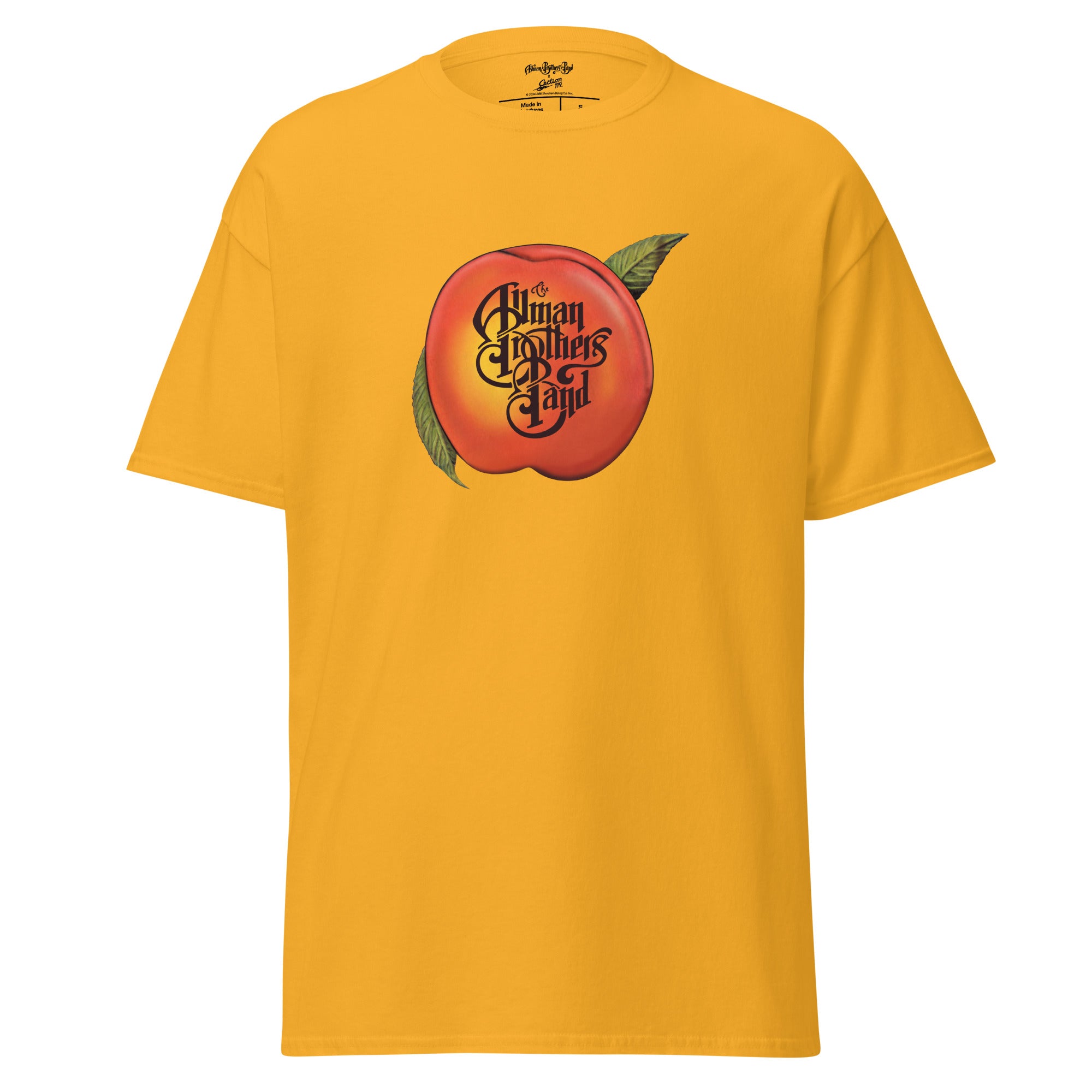This product photo features a bright yellow-orange T-shirt designed to promote the Allman Brothers Band. Set against a clean, white background, the shirt appears to be draped on a form, giving it a fitted look rather than lying flat. The T-shirt boasts a round neckline and short sleeves, with a straight waist design common in standard T-shirt styles. Dominating the front of the shirt is an eye-catching graphic of a peach with a green leaf curling around the bottom left and another leaf pointing out from the top right. Embedded in the peach graphic is the name "Allman Brothers Band" in a decorative black font, with the initials stylized in larger, swirling letters. The rest of the T-shirt remains plain, emphasizing the central design. The label at the back of the shirt is visible but unreadable, and the specific size and brand remain unidentified.